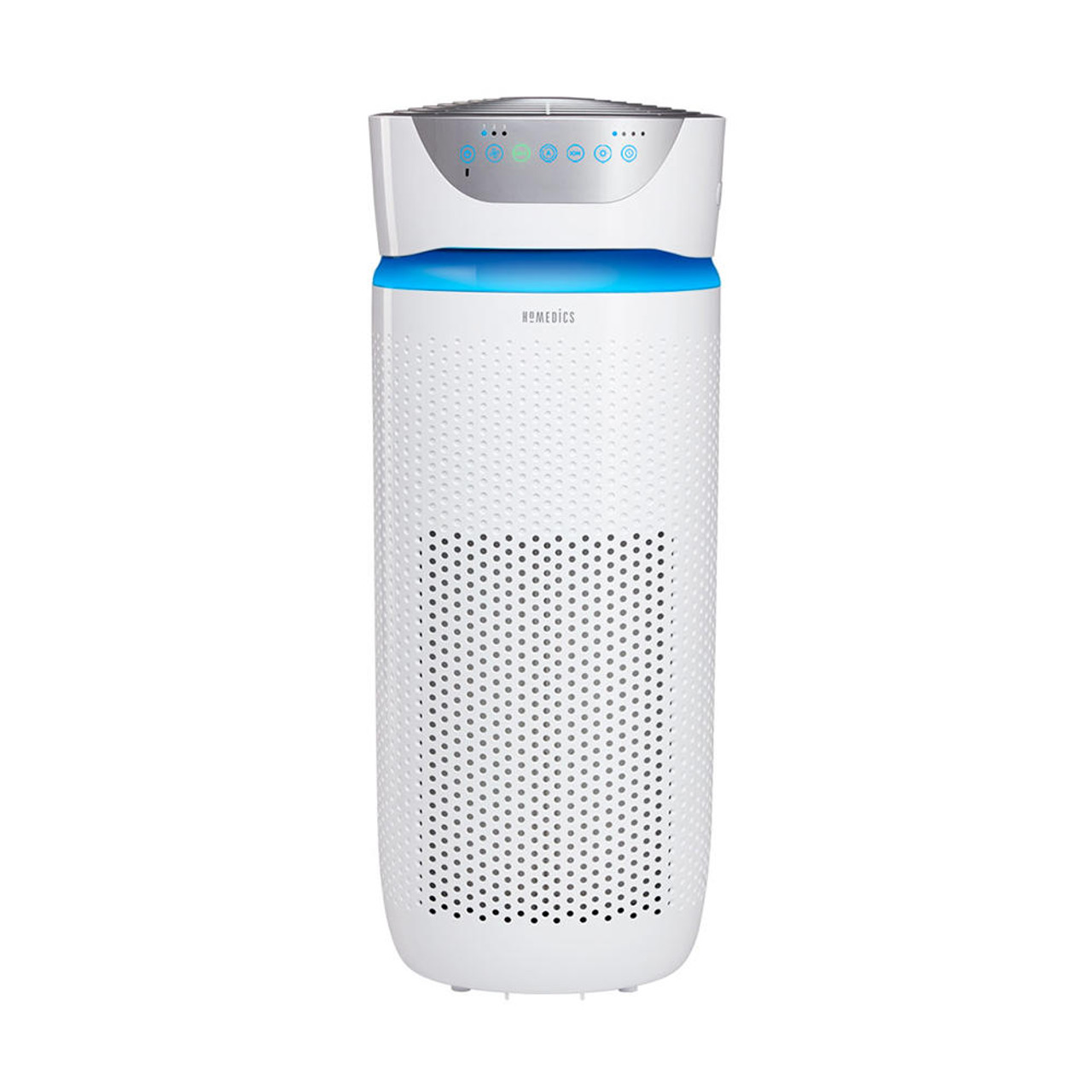This image showcases a streamlined air purifier or humidifier (possibly a fan or other air control device) made by Homedics. The device is primarily white with gray text, featuring the brand name "Homedics" prominently displayed towards the top. The device is taller than it is wide and has a grill composed of numerous small circles at the front, allowing air to flow through. Around 90% of the device is white, while the top 10% features a blend of white and silver, with a distinctive blue neck separating these two sections. Above the grill, there is a control panel with various buttons in blue and green, some of which are illuminated. The product is photographed against a plain, transparent background, ensuring the device is the focal point.